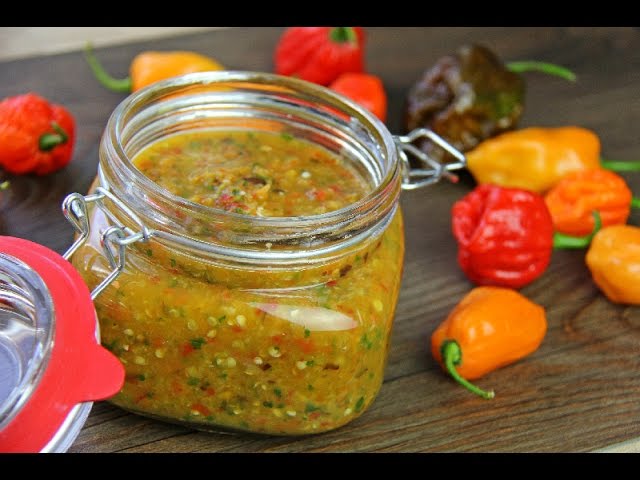The image features a short, ornate glass jar filled with a thick, vibrant spread or salsa. The jar is open, showcasing its rich, orangey-yellow contents speckled with green, red, and yellow bits. The jar has a distinctive sealing mechanism with a red, plastic seal and silver clamps to secure the top. Surrounding the jar on the wooden table are an array of colorful peppers—orange, red, dark green, yellow, and purple—all with green stems. Notably, one orange pepper appears shriveled and aged. The wooden table’s grain adds a rustic touch to the scene, highlighting the natural elements of the setting.